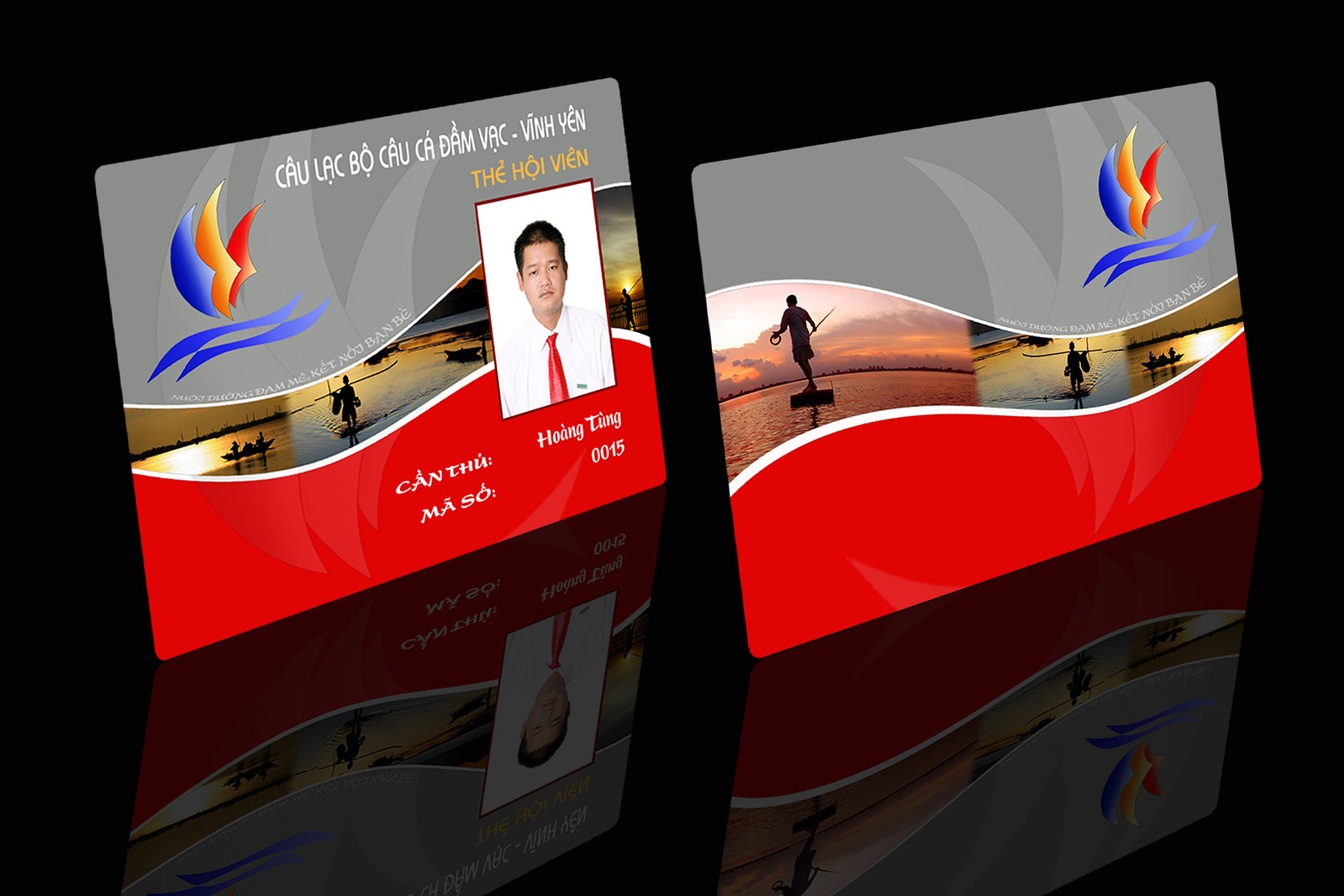The image showcases the front and back of a club card, displayed upright on a glossy black reflective surface, allowing the cards' reflections to be clearly seen. The cards, designed in shades of gray and red, feature a wave pattern with gray above and red below. In the center of the wave on the front card, there's a picture of a young Asian man dressed in a white shirt and red tie. Below the image, his name and the number '0015' are printed, with additional writing next to his name. Above the man's photo, the text "Hoi Vien" is visible, likely the club's name, written in a foreign language. The top portion of the card's gray background displays an emblem resembling blue, yellow, and red sails with two blue waves below. The design also includes imagery of people boating or fishing within the wave pattern. The card on the right appears to be the back side, identical in design but lacking the photograph and text.